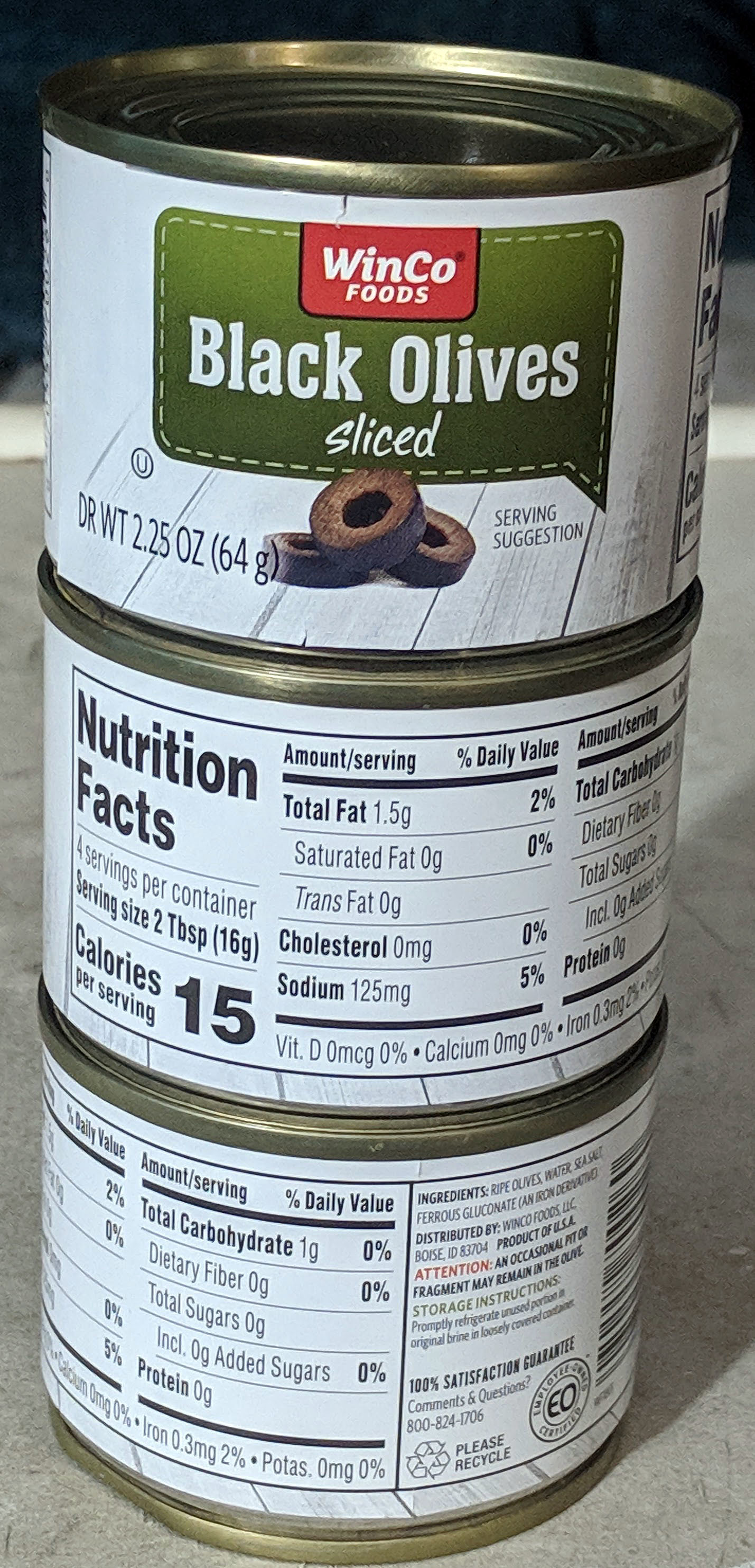This close-up photo showcases a neatly stacked trio of small tin cans containing sliced black olives. Each can features a predominant white label encircling the entire surface. The topmost can prominently displays the front label which includes a green speech bubble highlighting "Black Olives Sliced" in white text, accompanied by the red WinCo Foods logo at the top of the bubble. Just beneath this label, there is a clear, appetizing image of three black olives.

The middle can in the stack reveals the detailed nutrition facts, printed in black text against the white backdrop, providing essential dietary information. The bottom can, similarly, shows more nutritional data and additional product information in black lettering on the white label. The entire composition effectively displays various parts of the product's labeling, offering a comprehensive view of the packaging.